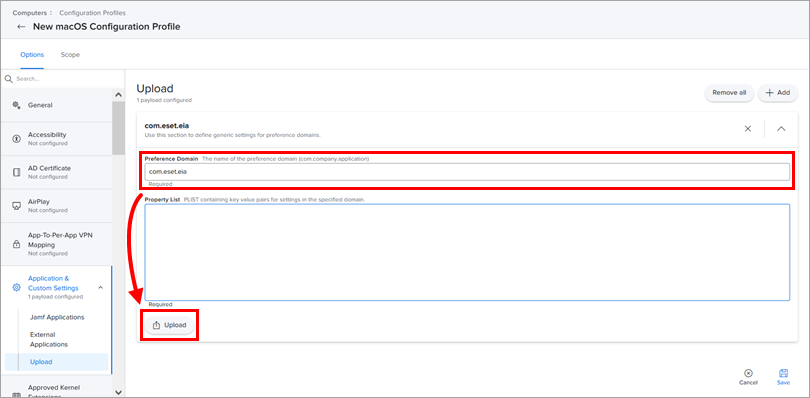Certainly! Here's a cleaned-up and detailed caption for the image described:

---

The image displays the settings section of a computer running macOS, specifically in the configuration profiles area. The interface is laid out with a dark theme, where primary headings are in bold black text. At the top, the section title reads "New macOS Configuration Profile," and underneath, there are various subsections. 

The "Scope" section is highlighted in blue, indicating it is currently selected or active. Below "Scope," there are multiple other options listed sequentially: General, Accessibility, Certificate, Add Play App, VPN Mapping, Application, Custom Settings, JMF Applications, External Applications, and Upload. 

In the center of the screen, a smaller section includes buttons for "Upload" and "Add," with a corresponding "Remove All" option. Red text highlights point to areas that might need user attention, and a downward-pointing arrow is labeled "Upload" near a search bar. Below this central part, there's a comment section labeled "Property List."

At the bottom right corner, there are two action buttons: "Cancel" and "Save."

---

This detailed and structured caption gives a clear representation of the interface and the various elements within the image.